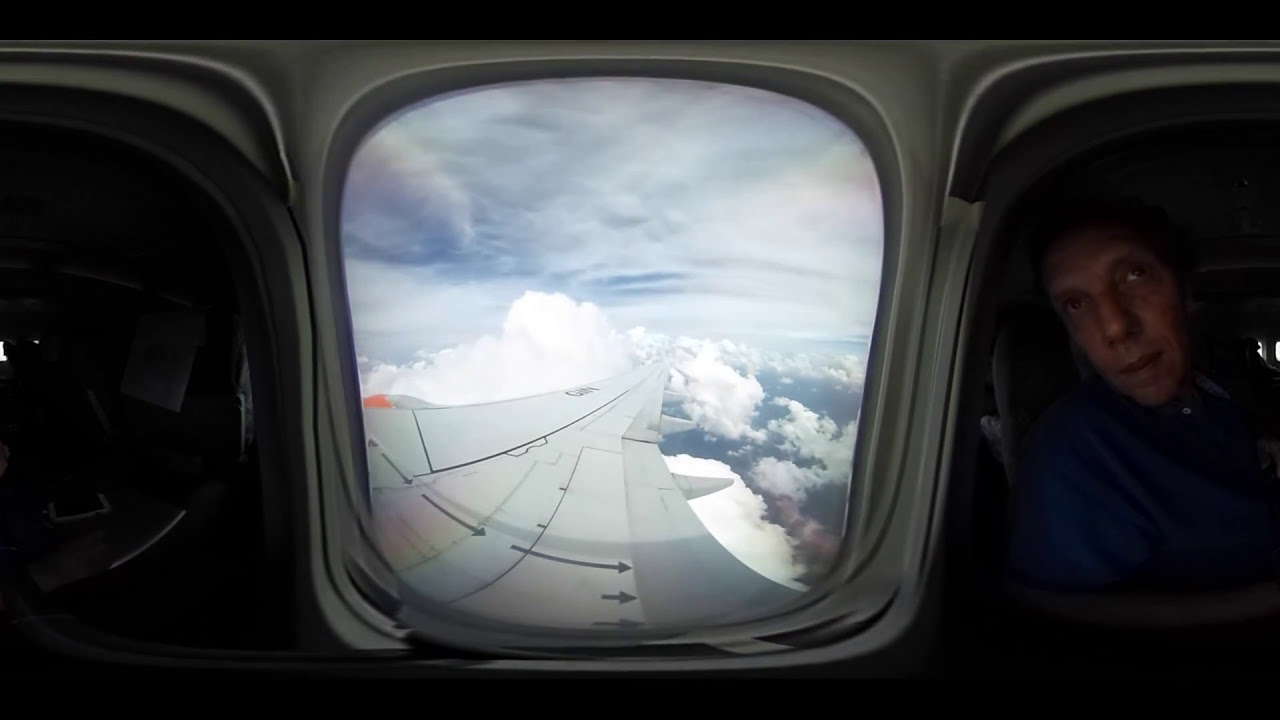The image is framed with a thin black border along the top and bottom, and features three distinct sections resembling airplane windows, surrounded by a gray casing. The left window exhibits a dark interior view of the airplane, where a couple of airline seats are faintly visible. The middle window presents a reversed perspective, looking out from inside the airplane at a wing emblazoned with a small red mark, possibly the plane’s logo, extending into a sky filled with clouds. Beneath and above the wing, patches of blue sky and clouds indicate daytime flight, with the ground faintly discernible below the clouds. The right window offers another view inside the airplane, where a white male wearing a dark blue long-sleeve shirt is seen looking out and slightly up to his left, his mouth closed, not directly facing the camera. Additionally, there are arrows pointing to the right beneath the windows, with three long arrows and two shorter ones underneath.